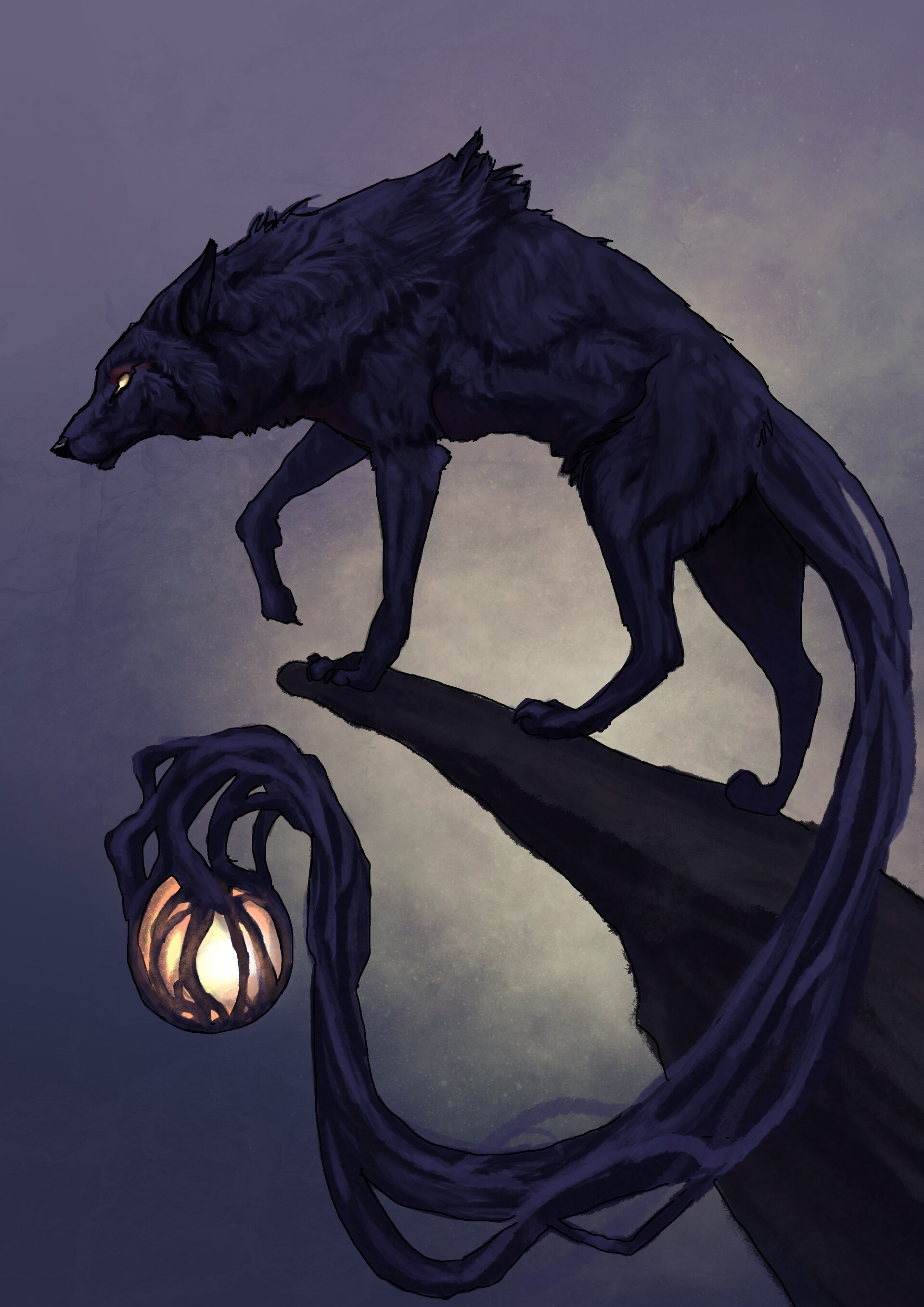The image portrays a shadowy, purple-toned wolf-like creature standing dramatically on the edge of a narrow, brown cliff. This fantastical beast, with ragged fur and black accents, has an eerie, ghost-like tendrilled tail which wraps around and grasps a glowing yellow orb. The wolf has piercing yellow eyes and stands on three legs, its fourth paw lifted and pointed inward, creating a dynamic stance. The background features a cloudy, purplish and dark blue sky with lighter tones toward the center, emphasizing the ethereal, otherworldly presence of the wolf. The creature's back hair stands on end, adding to its ominous and mystical aura.